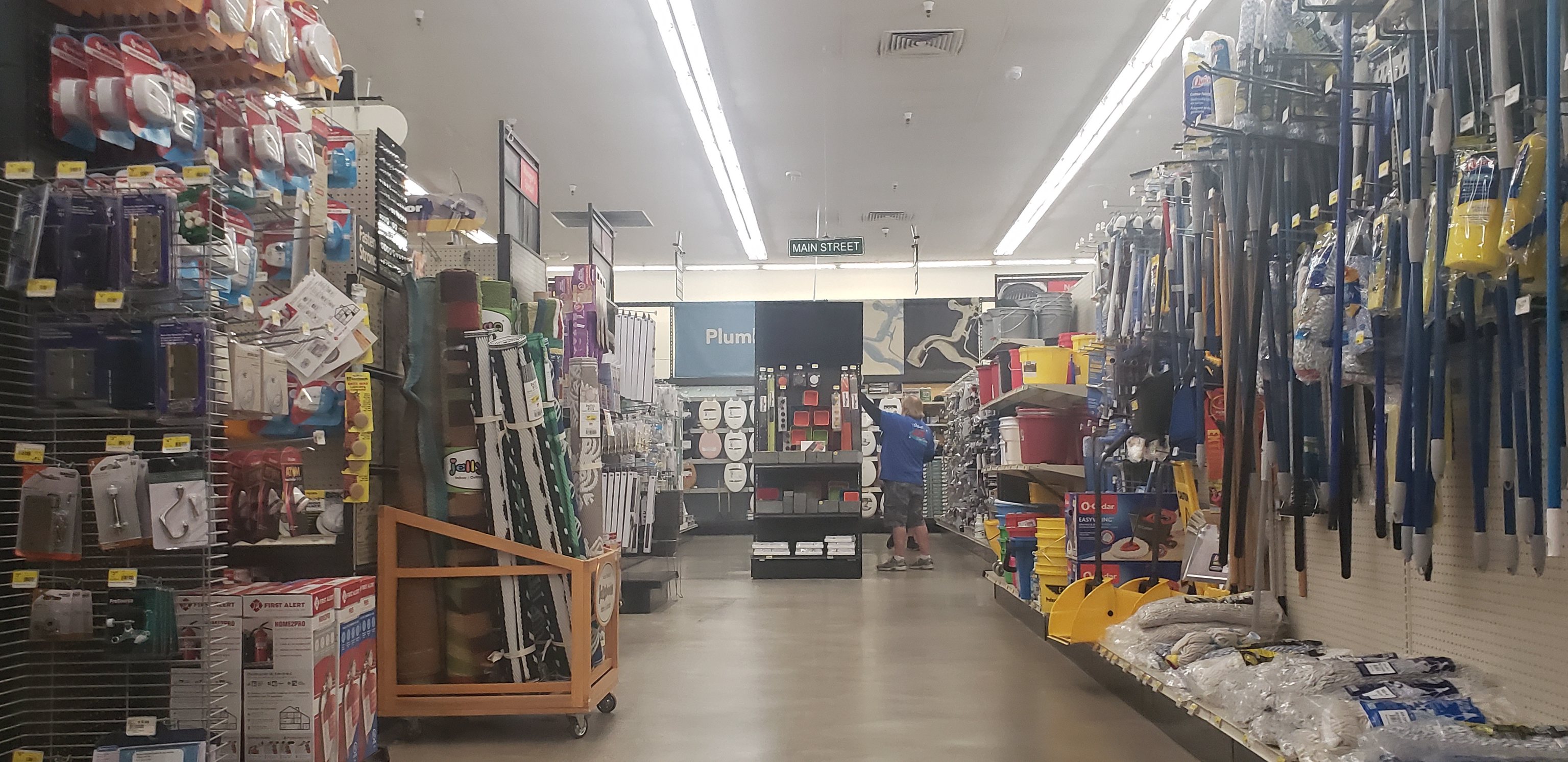This detailed image captures the interior of a hardware store, specifically focusing on a walkway between two rows of aisles. On the left-hand side, the aisle is displayed horizontally along the length of the wall, showcasing a full view of an assortment of tools and supplies neatly organized for customer browsing. The right-hand side features an aisle adorned with various wooden handles, possibly for tools such as hammers, rakes, or brooms. Additionally, the lower portion of this aisle holds a bag containing a substance, suggesting items like potting soil, concrete mix, or another commonly used material in hardware projects. The overall layout and abundant product offerings reflect a well-stocked and meticulously arranged hardware store aisle, inviting customers to explore and find everything they need for their DIY projects.